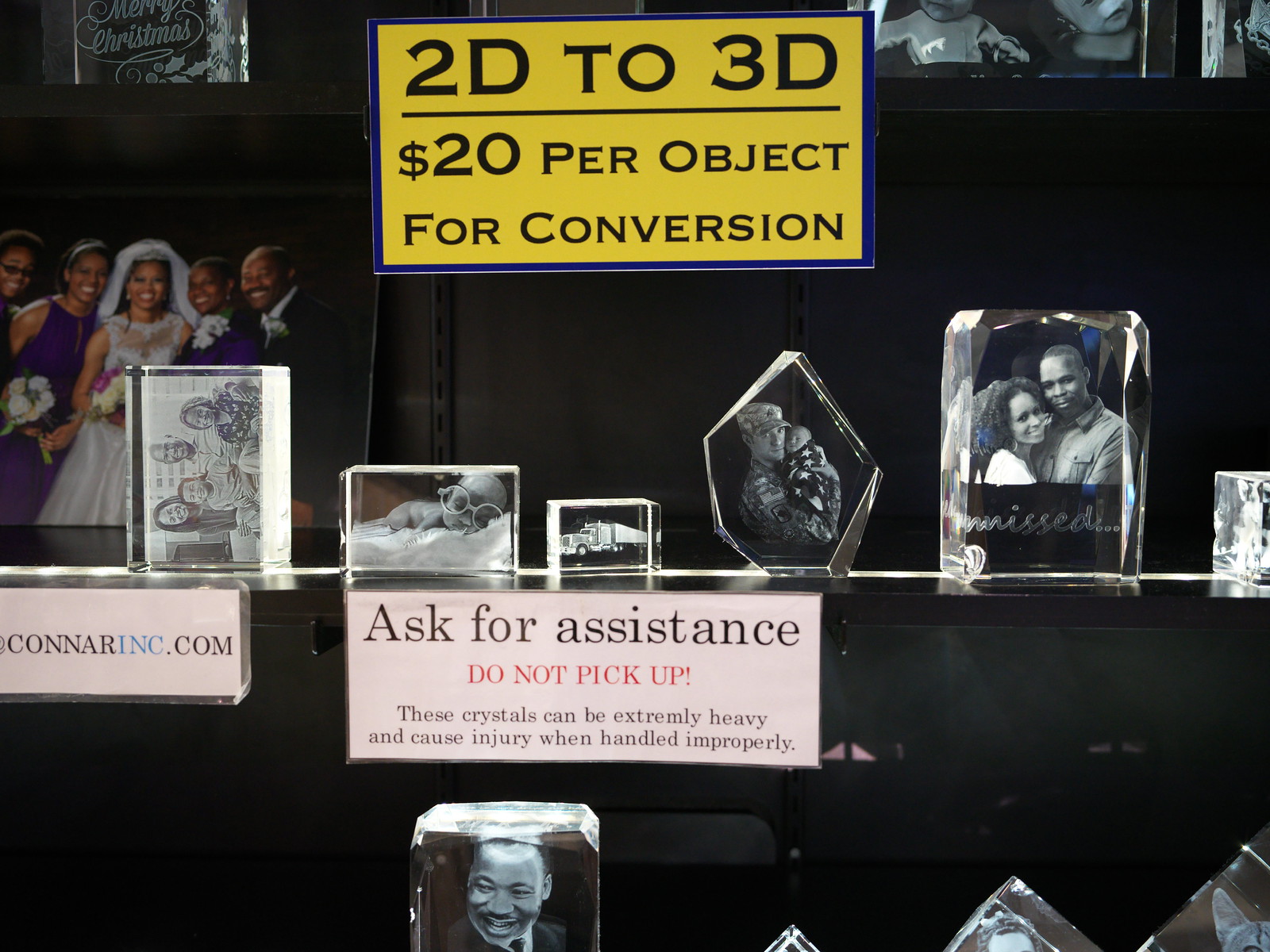The image showcases shelves adorned with an assortment of decorative crystals, each embedding a photo. Prominently displayed is a yellow sign with a blue border and black text that reads, "2D to 3D, $20 per object for conversion." Below it, a small white sign cautions, "Ask for assistance, do not pick up. These crystals can be extremely heavy and cause injury when handled improperly." Another sign advertises a website, connorinc.com.

The crystals come in various shapes and sizes, including vertical and horizontal rectangles and diamond-like forms. Each crystal features detailed engravings of diverse subjects: a soldier holding a baby, a portrait of Martin Luther King Jr., a truck, a couple, a "Merry Christmas" inscription, a wedding photo, and a family photo. The entire scene vividly captures the transition from 2D images to 3D crystal engravings, highlighting both the artistic and functional aspects of these unique keepsakes.